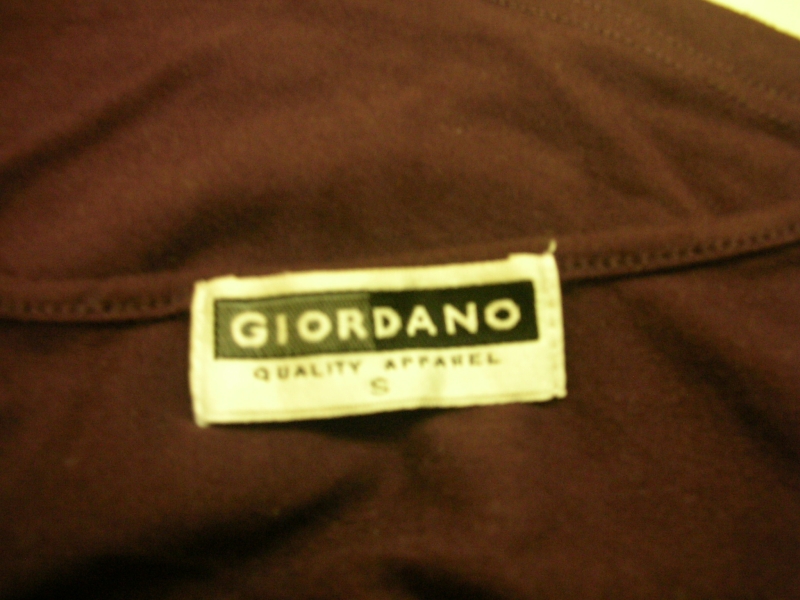This image captures a close-up view of the back tag on a piece of clothing, specifically a black garment that could either be a shirt or sweater. The fabric appears slightly faded, giving it a grayish tint. Detailed stitching is visible along the left and right sides of the fabric. The focal point of the image is a rectangular, yellow tag centrally positioned. The tag displays the brand name "G.R. Daniel" prominently at the top, with "Quality Apparel" written underneath. At the lower part of the tag, the size is indicated as "S" for small. In the upper right corner of the image, part of the yellow background peeks through, adding a contrasting element to the scene.